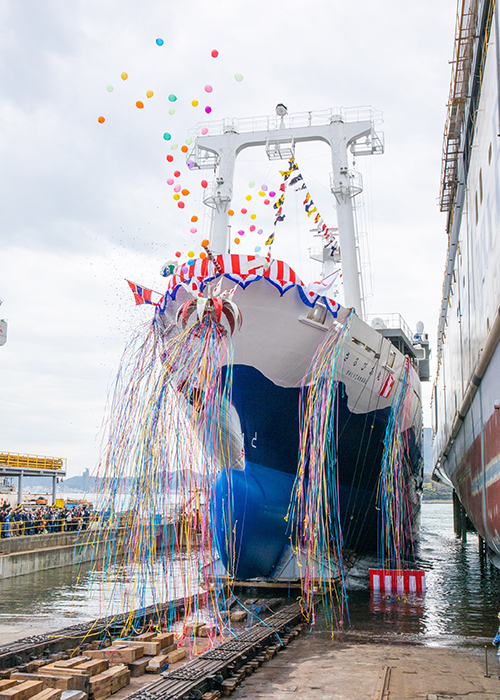This vibrant vertical portrait captures the celebratory launch of a new ship. The ship itself features a striking blue lower half and a pristine white upper deck adorned with an array of colorful streamers. Rainbow-colored streamers cascade down from the antenna tower and deck, draping gracefully over the ship. On the bow, red, white, and blue bunting adds to the festive atmosphere. The large white archway at the top of the ship also supports more streamers.

In the center of the image, multicolored balloons—red, pink, yellow—soar into the cloudy, hazy gray sky, marking the joyous occasion. The harbor's water below is a murky light brown to dark green. On the left side of the image, a distant crowd gathers on the dock, which is separated by a yellow railing. The dock itself extends into a concrete sidewalk area with rows of bricks and a few crates visible.

This image encapsulates the momentous launch of the ship, possibly its inaugural voyage, complete with a diverse assemblage of festive decorations and an atmosphere brimming with anticipation and celebration.